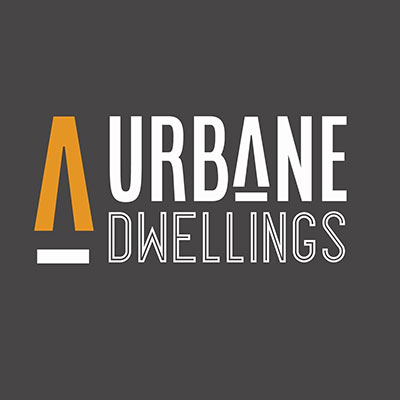The image depicts a dark gray square background featuring prominently in the middle. On the left, there is an upside-down orange V resembling a tent, with a white line under it, forming a logo-like symbol. Adjacent to this on the right is the word "URBANE," in bold, all-capital white letters. The 'A' in "URBANE" mirrors the logo with an upside-down V and an underlining bar. Beneath "URBANE" is the word "DWELLINGS," written in outlined white letters with a dark gray filling, smaller in size compared to "URBANE." This image, with its professional and minimalist design, closely resembles a business card or a logo for a brand named "Urbane Dwellings."